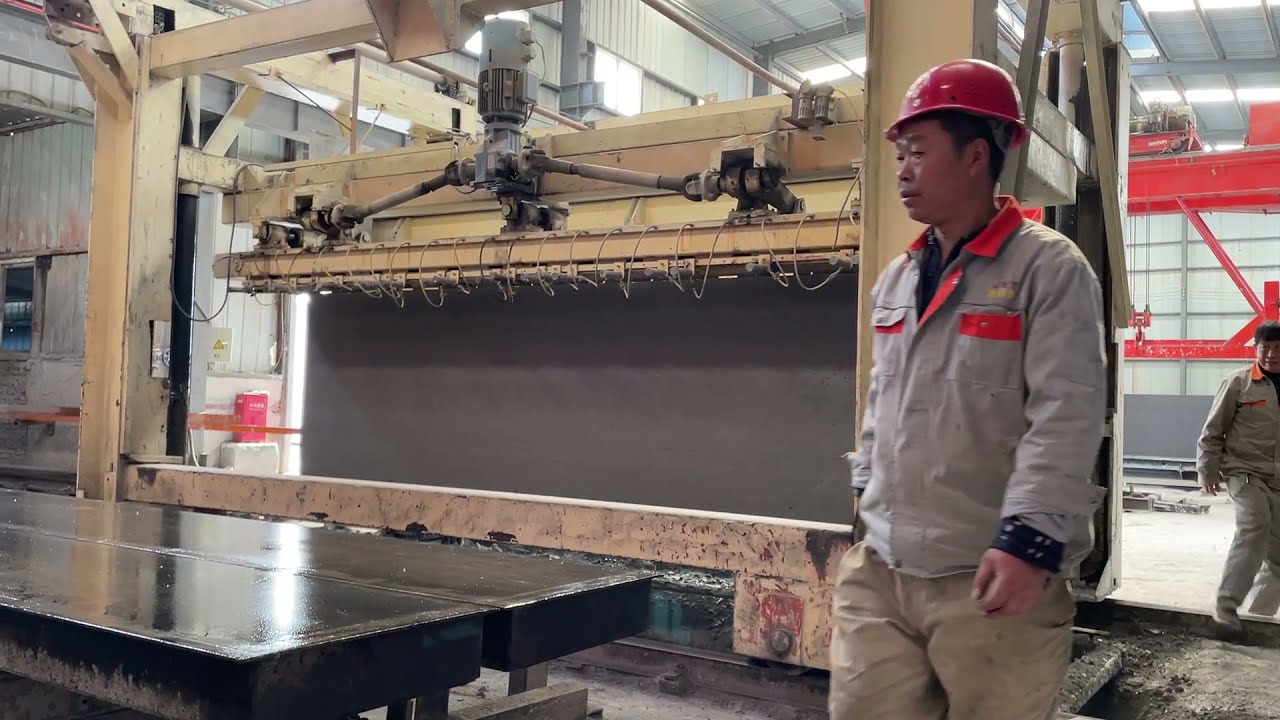In the photo, a factory worker clad in a red hard hat stands poised next to a large, black work table with a shiny surface. He is dressed in beige khaki pants and a gray zip-up jacket accented with a red collar and red pockets. The industrial setting behind him features high-rising red ladders, well-worn tan machinery with bars extending across, and windows that let in ample light, illuminating the factory's gritty ambiance. Dirt and grime coat much of the yellow industrial equipment scattered around the room. Another worker, in a similar uniform but without a hard hat, stands in the background, observing the scene. The environment suggests active industrial production, possibly involving spray paint or similar materials, underscoring the facility's role in manufacturing.